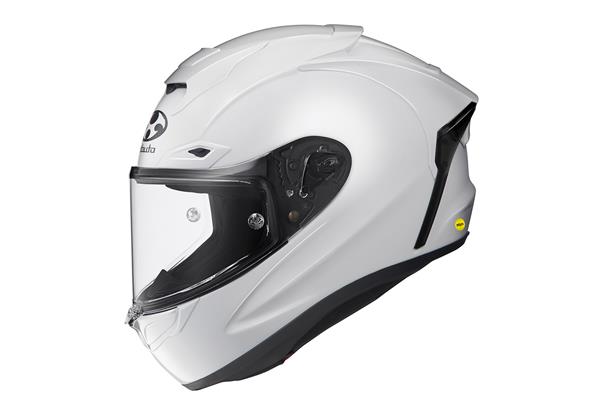This image depicts a sleek and modern motorcycle helmet, dominantly white with black accents and a clear visor. The helmet, featuring a mix of futuristic and contemporary design elements, is facing to the left on a plain white background. The helmet's appearance is enhanced by a partial logo above the visor, which seems to end with the letters "D-A" and contains a circular emblem with a ninja throwing star design. It also has a yellow sticker with black writing on the bottom right side. The helmet is well-ventilated with noticeable vents at the front and potential vents at the back, highlighted in black, which add to its safety features. The clear visor, which can be raised, offers practical usability for different riding conditions. The interior padding, visible through the clear visor, is black, complementing the helmet's overall aesthetic. This sophisticated helmet, showcasing a blend of white and black hues, is not only visually appealing but exudes an aura of safety and protection.